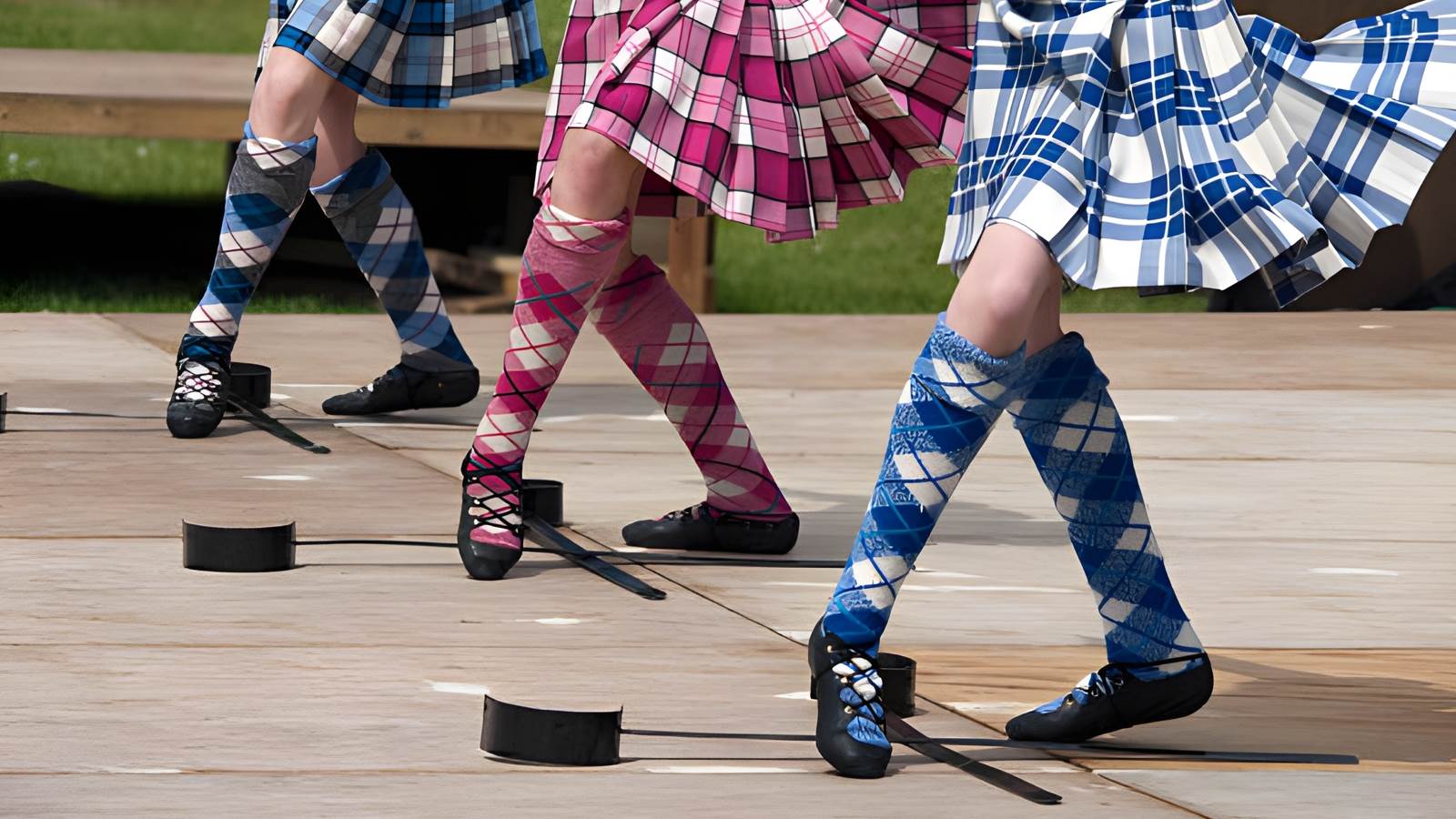The image features three individuals, each sporting checkered skirts and matching socks, with the scene captured from the waist down. The person at the back dons a bright blue skirt with navy blue and white plaid stripes, complemented by white and blue plaid socks. Moving forward, the individual in the middle wears a magenta skirt exhibiting white checkered patterns, along with magenta plaid socks. The frontmost person is clad in a white skirt adorned with royal blue checkered markings, paired with matching socks and black shoes. The setting includes a light brown concrete ground, a light brown bench, and patches of green grass. Notably, the individuals' positions and outfits suggest they might be dancers, given their coordinated attire and slightly angled ankles.